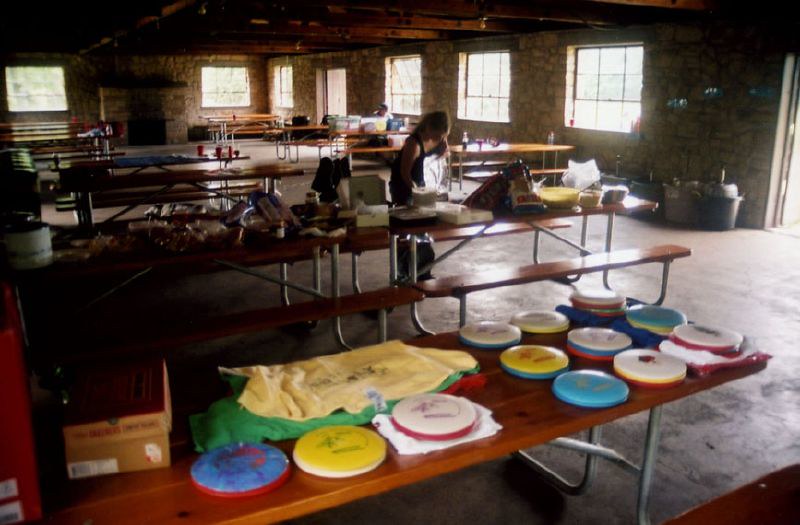The photo captures a spacious, dimly-lit room, possibly within a summer camp building, characterized by its concrete floor and rocky-looking walls. Sunlight streams through numerous large square windows lining both the left and right walls, with one window framing a distant fireplace. An open door lets light spill into the room, emphasizing its large, open atmosphere. Within this room, wooden picnic tables and benches are arranged in rows; those closer to the camera are heavily laden with various objects including colorful frisbees, plates, cups, and cakes in hues of blue, white, red, and yellow. Centered in the frame, a woman with short hair, dressed in a black top with a strap over the shoulder, stands slightly hunched over, busy with an object on one of the benches. Additionally, among the scattered items, an open box and a yellow t-shirt atop a green one are prominently visible. The overall scene suggests a crafts or preparation area, possibly set up for an event involving customized frisbees and baked goods.